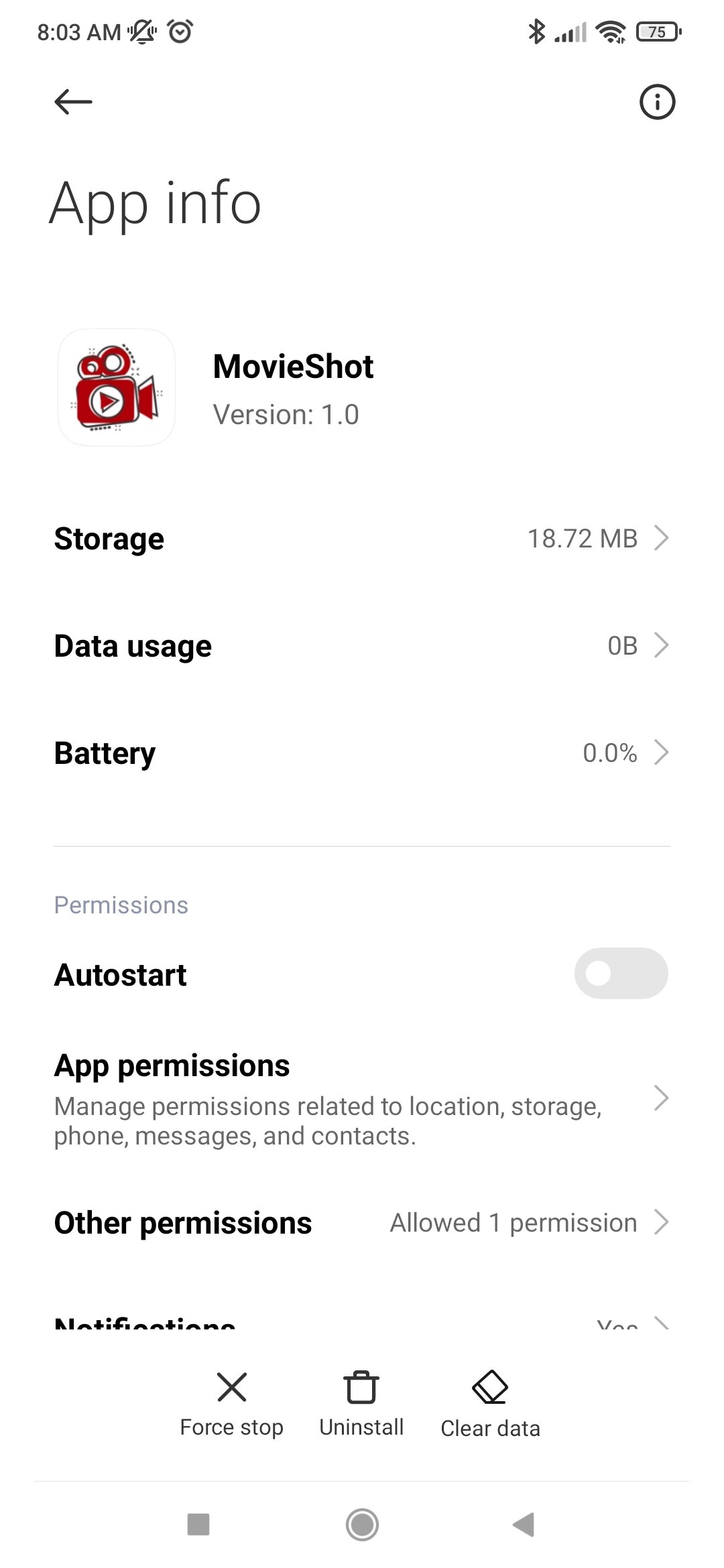The image showcases a screenshot from a mobile device, captured at 8:03 AM as indicated by the time displayed in the top left corner. The device's status bar contains several icons: a mute icon, an activated alarm icon, and a Bluetooth icon signalling that it is not connected. The network signal strength is shown at 3 out of 5 bars while the WiFi signal is strong at 4 out of 4 bars. The battery level is at 75%.

Below the status bar, the screen displays information about an application named "Movie Shot," version 1.0. Additional app details reveal that it has used 18.72MB of storage and currently has a data usage of 0 bytes. The battery usage by the app stands at 0.0%. Permissions are managed for the app, including auto start and one other permission. The application is granted permissions related to location, storage, phone, messages, and contacts.